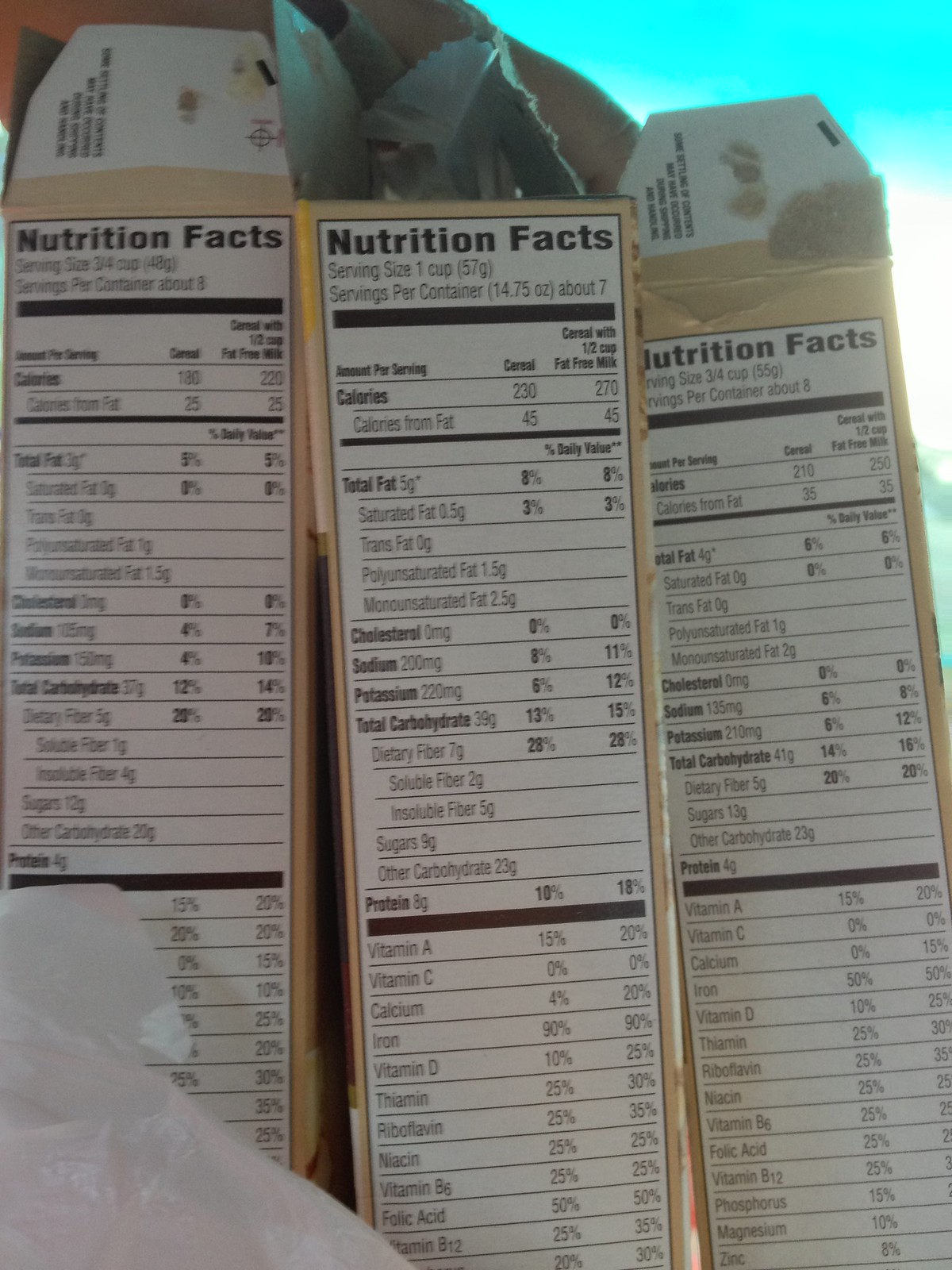The image features three identical tan-colored boxes, all oriented with their Nutrition Facts sides facing the viewer. Each box is structured with a white top flap and a distinct bright turquoise section in the top right corner. The leftmost box has a piece of grayish-white tissue paper obscuring the lower part of the vitamins section on the Nutrition Facts label. The middle and rightmost boxes also display comprehensive Nutrition Facts labels from top to bottom, with no obstructions. This composition provides a clear view of the nutritional information, highlighting minor packaging variations across the three boxes while maintaining a uniform overall appearance.